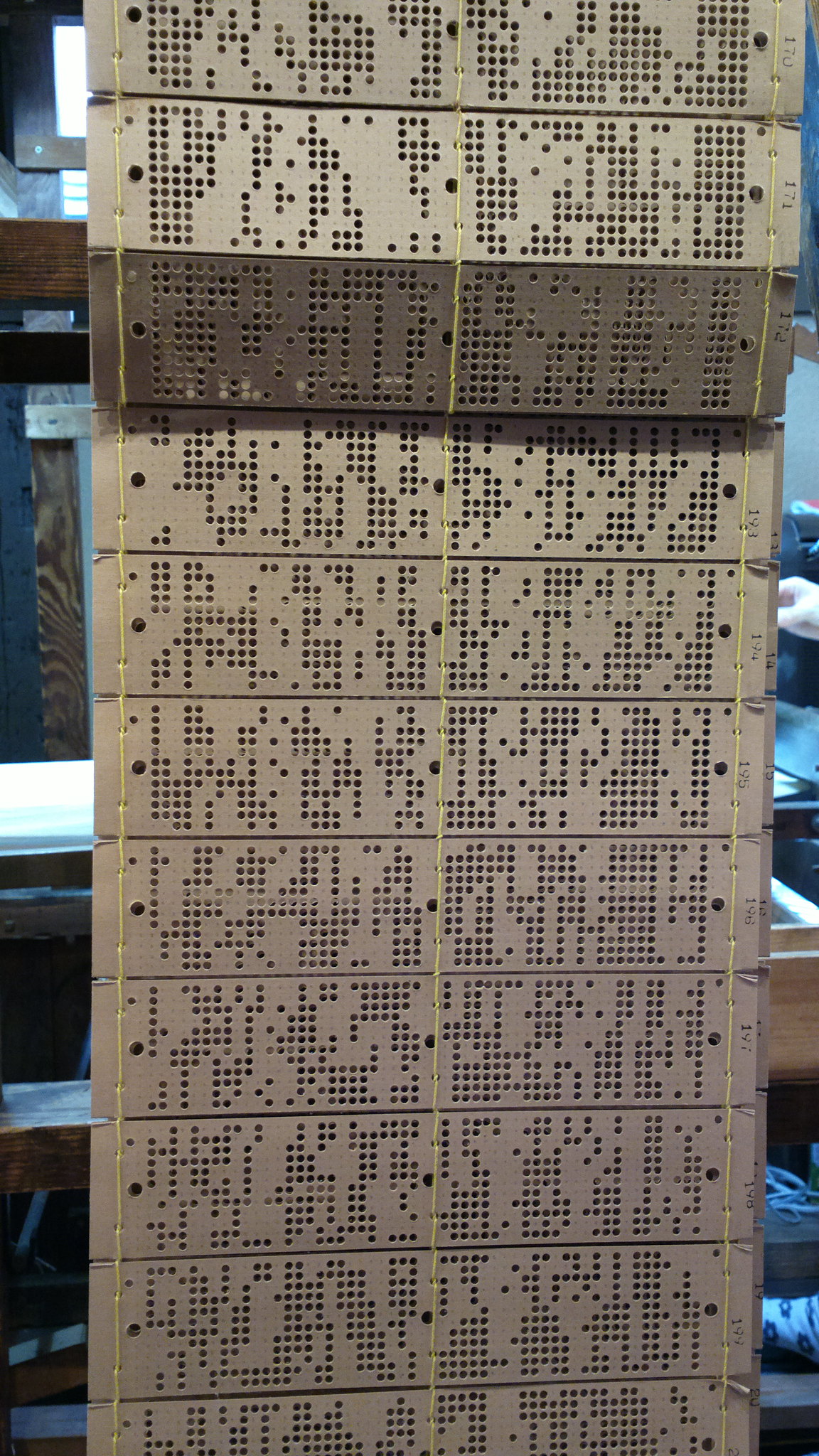The photograph captures a peculiar object that consists of several long, narrow panels, draped vertically from the center top to the center bottom of the image. These panels, resembling ruler-sized pieces of wood or potentially thin metal, feature numerous deliberately punched holes arranged in varied patterns. The panels are predominantly light tan in color, except for the third one from the top, which stands out with a dark brown hue. Each panel is interconnected using stitching made of thin, neon yellow string, with connections visible on the left side, right side, and center. Distinct dark writing runs horizontally across the panels. 

In the background, the object appears to be positioned in front of a bookcase or shelving unit filled with an assortment of dark and light items. Additional background details include visible wood grain on the left side and what seems to be a hand in the top middle area, accompanied by a piece of clothing with floral patterns at the bottom right. The object's material and purpose remain ambiguous, contributing to its bizarre and intriguing appearance.